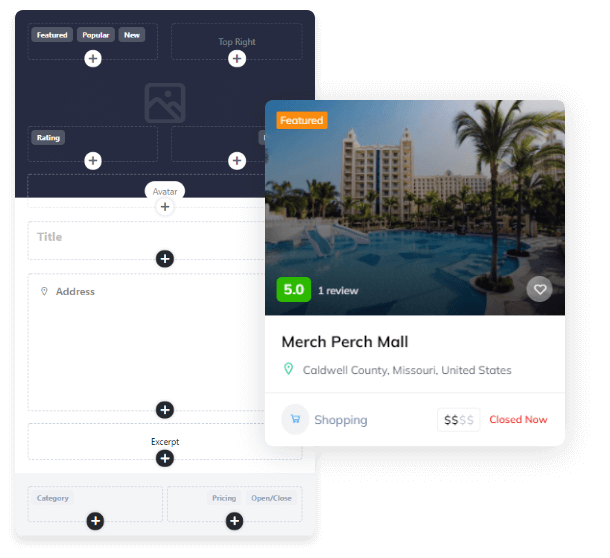This image appears to be a composite of two distinct sections, potentially sourced from a web application interface. The lower section is characterized by a series of interactive UI elements. It includes a set of buttons labeled "Featured," "Popular," and "New," all contained within a dotted rectangular frame. The “Featured” button is visually highlighted with a grayish, oval shape.

Within this frame, there are four additional rectangular segments arranged in a 2x2 grid. Each of these segments is marked by a white circle with a white plus sign at their bottom center, suggesting the option to add or customize content. Nestled between these segments is an icon representing an image, set against a dark blue background.

Below this primary section, another feature area is visible. This includes a central label reading "Avatar" with an accompanying circle containing a plus sign, likely indicating a profile picture upload or selection button. Just below, there is a rectangular field labeled "Title." Further down, there’s another interactive element—a black circle with a white plus sign—followed by fields labeled "Address" and "Excerpt," suggesting input areas for textual information. To the right of these fields, two buttons labeled "Category" and "Pricing" provide additional functional options.

On the right side of the image, there is a depiction of what seems to be a listing or product card. This section features an image banner with the text "Merch Perch Mall" and a five-star rating based on one review. The top of this card displays the label "Featured," underscoring its importance or highlighted status within the interface.

Overall, the image presents an intricate and detailed interface layout with multiple interactive elements and content segments designed for user interaction and content management.